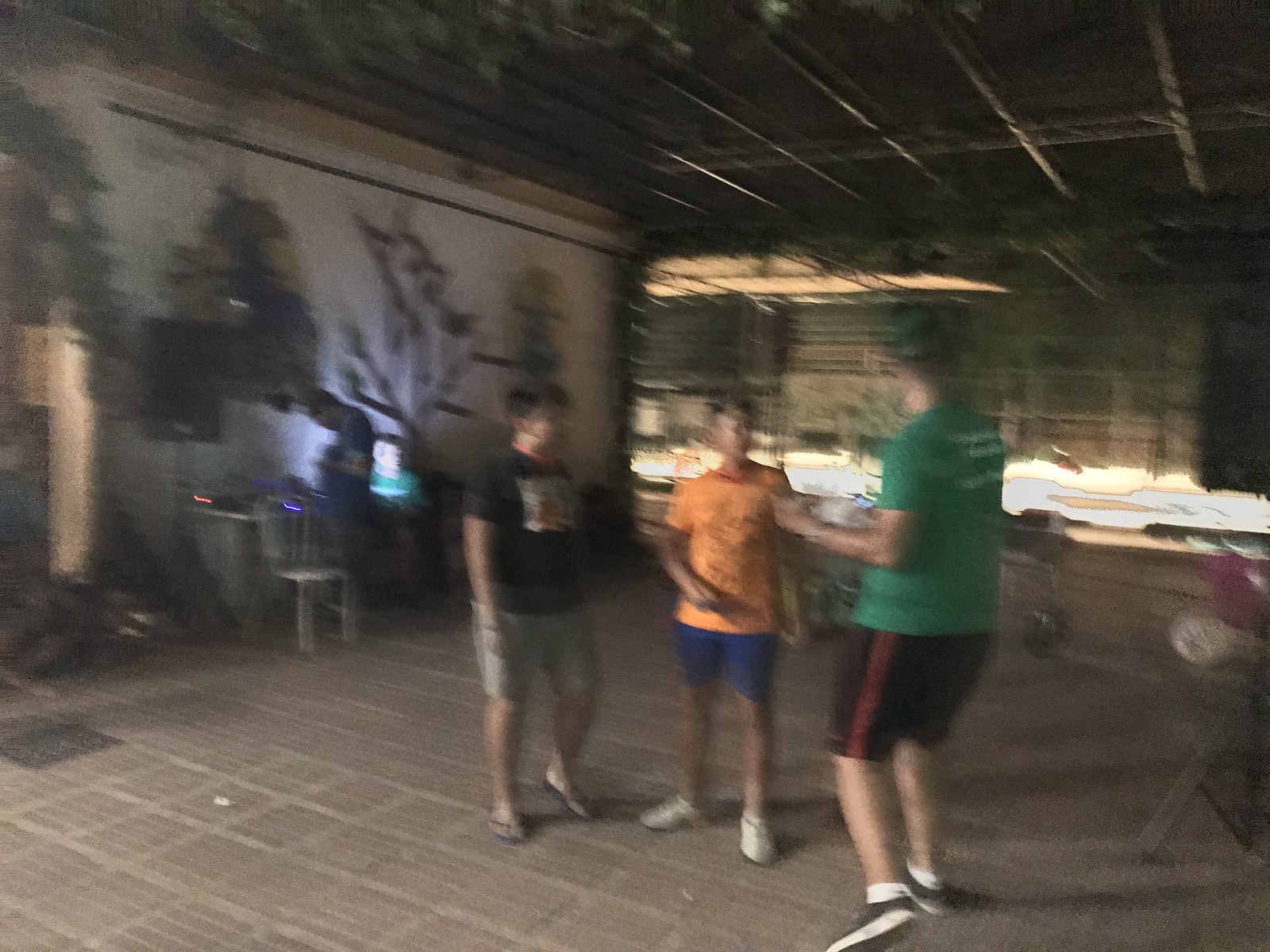A blurry photograph captures three individuals engaged in conversation, each clad in shorts of different colors. The tallest among them, wearing a green shirt and black shorts, stands slightly apart from the other two, who are of similar height. One dons an orange shirt with blue shorts, while the third sports a black shirt adorned with a design and paired with gray shorts. The setting is somewhat ambiguous but features a visible chair, a desk-like structure, and a floor covered in tiles, providing a casual backdrop to their interaction.